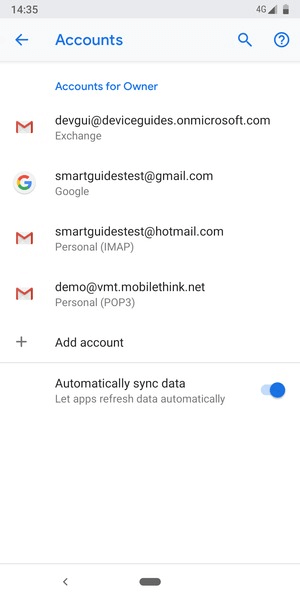The image depicts a smartphone screen displaying the "Account Settings" page. The time shown on the top left corner is 14:35, along with grey icons for battery and 4G network strength located at the top right corner. The background at the top is light grey, while the main page background is white.

The title "Accounts" is prominently displayed in blue, accompanied by a blue back arrow on the left and a blue search icon and help icon on the right. The help icon is depicted as a blue question mark inside a circle.

Below the title, there's a section labeled "Account for owner" also written in blue. This section lists several accounts:
1. The first account, an Exchange account, is "devguidesdeviceguides.com on microsoft.com," marked with the Microsoft icon—a white envelope with a red "M."
2. The second account, "smartguidetest@gmail.com," is a Google account represented by the multicolored "G" icon in red, yellow, green, and blue.
3. The third account, another Exchange account, is "smartguidetest@hotmail.com," labeled as "personal IMAP."
4. The fourth account, also an Exchange type, is "demo@VMTmobilethink.net," labeled as "personal POP3."

At the bottom of the page, an "Add account" button is visible. Below this, there's a toggle switch for "Automatically sync data," described with the text "Let apps refresh data automatically." The switch is toggled on, indicated by its blue color on the right side.